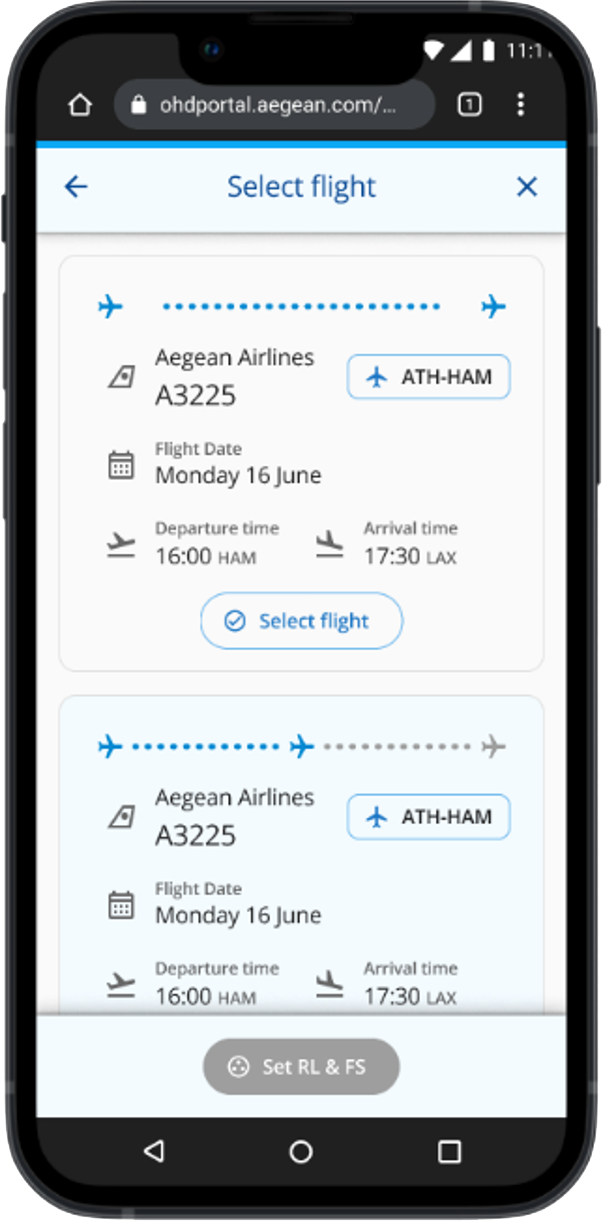The image displays a mobile phone screen showing a flight selection interface on the odportal.aegn.com website. Below the website's address bar, there is a white box with the text "Select Flight" in blue, accompanied by a blue arrow on the left and a gray X on the right. 

The main section consists of a gray background featuring a sequence of small blue airplane icons moving across the screen from left to right, symbolizing the flight journey.

Flight details are provided for two segments:
1. **First Segment:**
   - **Airline:** GN Airlines
   - **Flight Number:** A3225
   - **Departure:** Monday, June 16th, 4:00 PM from Hamburg (HAM)
   - **Arrival:** 5:30 PM at Los Angeles (LAX)

2. **Second Segment:**
   - **Route:** Athens (ATH) to Hamburg (HAM)
   - **Flight Number:** Not specified
   - **Departure:** 4:00 PM (1600)
   - **Arrival:** 5:30 PM (1730) at Los Angeles (LAX)

An explanation clarifies that the traveler must first fly from Athens to Hamburg to connect to the Hamburg-Los Angeles flight. 

Each segment includes a button labeled "Select Flight" for booking selections.